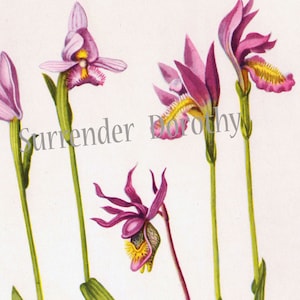The image is a square, multi-color artistic print of five distinct flowers against a light purple background. The flowers have thin green stems with leaves positioned towards the middle and top. The petals are predominantly purple, displaying a range of orientations with some petals extending horizontally while others extend vertically. Intricate, yellow silicate hairs emerge from the center of each flower. Notably, one flower towards the center is positioned lower than the others.

Overlaying the image, a grey text reading "Surrender Dorothy" spans across the center of the picture, serving as a watermark or label. The stem of the central flower appears reddish or pink and falls just below this grey text overlay. The detailed petals of the flowers are eye-catching, with some petals featuring hints of magenta at their edges. The inclusion of the "Surrender Dorothy" text, though referencing the Wizard of Oz, adds an unexpected digital element to this artistic portrayal of peculiar, vividly colored flowers.